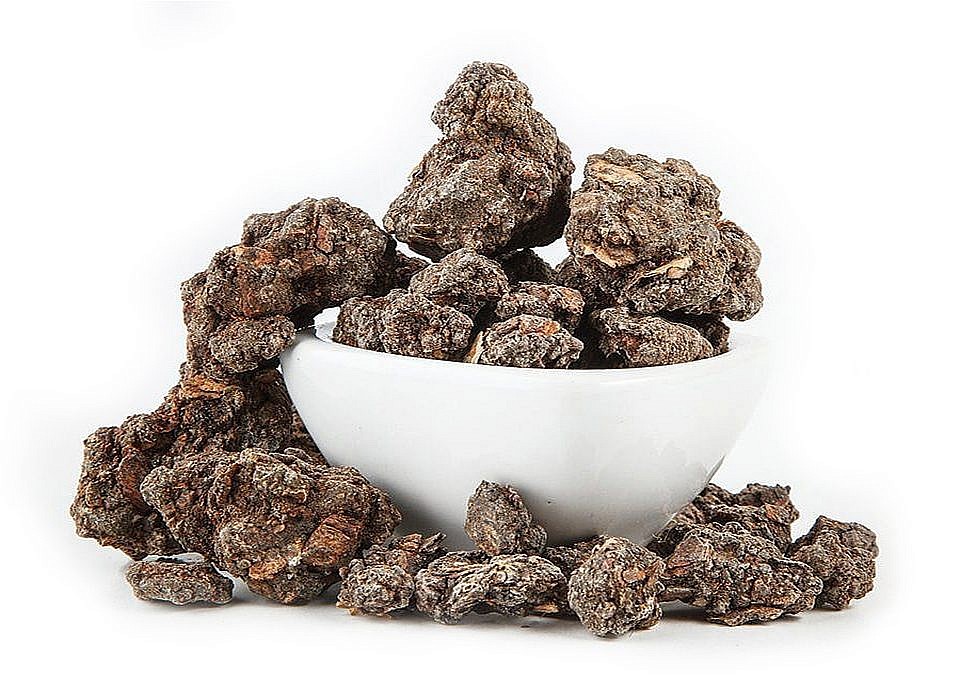In the center of a pristine white background, a small white ceramic bowl is prominently featured, likely from a sales website or stock product image. The bowl, filled to the brim with a collection of variously sized stones, is overflowing, with the stones cascading down the left side and scattered around the base on the white surface it rests on. The stones, predominantly brown with reddish portions, also possess shades of greenish-gray, presenting a natural, earthy palette. The stones are irregular in shape, ranging from long to small, with the largest piece notably positioned upright at the center of the bowl. Shadows cast by the stones add depth to the image, suggesting a light source from the front. The detailed arrangement and diverse textures suggest the stones could be mistaken for covered nuts or truffles, adding an element of intrigue to the overall composition.